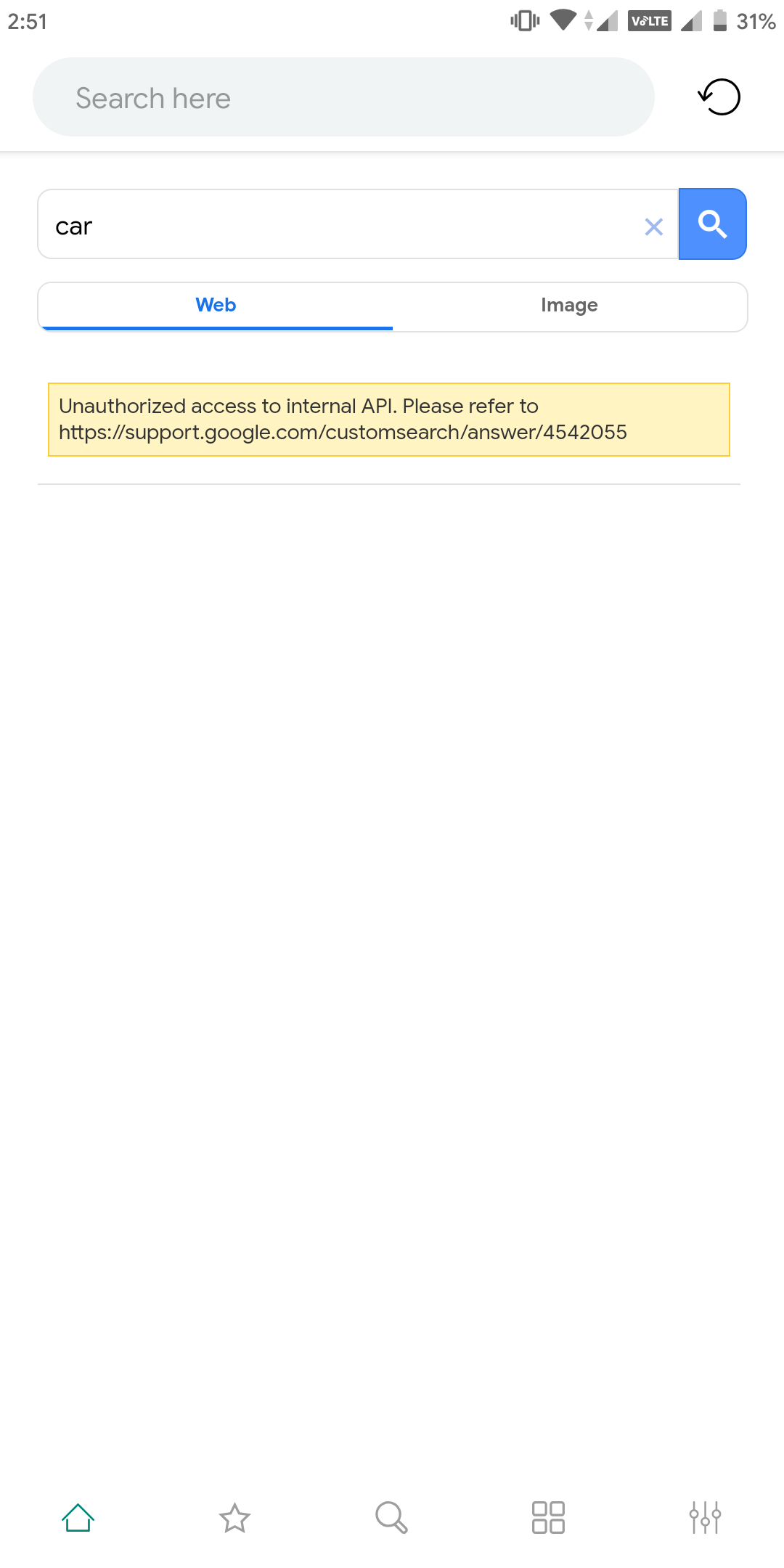This image is a detailed screenshot captured from a smartphone. At the very top, an open search bar can be seen, with the placeholder text reading "Search here." Adjacent to the search bar on the right side is a reload button. The time displayed in the top left corner indicates it is 2:51 PM, while the battery icon on the top right corner shows a battery percentage of 31%.

Just beneath the search bar, there is a text entry field containing the word "car," followed by the word "blue." Below this, the screen is divided into two sections labeled "Web" and "Image." Immediately underneath, a prominent yellow box displays a warning message: "Unauthorized access to internet API. Please refer." This message is accompanied by a link to a website for further reference.

At the very bottom of the screen, five icons are neatly arranged: a home button, a star symbolizing favorites, a search button, a menu button, and a settings button. Back at the top, several other icons are visible, including the battery indicator, signal strength bars, and the Wi-Fi signal strength icon. The background throughout the image is a plain white negative space, which brings focus to the elements on the screen.